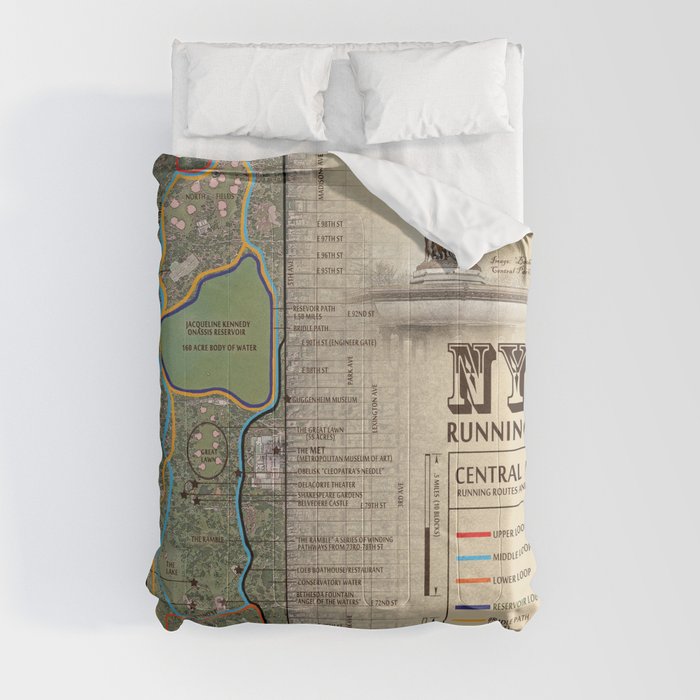In this top-down photograph, the focal point is a bed dressed in white sheets and adorned with two white pillows positioned at the head. The primary feature of the image is a puffy, thick quilted duvet or bedspread that showcases a detailed map design. The map, resembling a vintage aerial depiction of New York City's Central Park, spans the entire surface of the duvet. It is predominantly tannish in color with gray and green terrain indicating various areas within the park. Notable features on the duvet include the Jacqueline Kennedy Onassis Reservoir, a green landmass illustrating the Great Lawn, and numerous black lines denoting streets and pathways such as 88th Street, 97th Street, and Reservoir Path. Additionally, partial text on the right side of the duvet reads "NY" and underneath, it appears to say "running" framed centrally, hinting at "Central Park Running Routes." The duvet even lists different routes like the Upper Loop, Middle Loop, and Lower Loop. The upper right corner of the duvet is artistically turned down, revealing the white fabric underneath, further emphasizing the bed's sophistication against its stark white background.